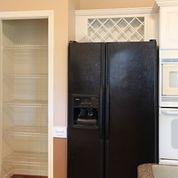This is a small, square-shaped, lower-quality photograph, likely taken inside a kitchen. The back wall of the kitchen is divided: the top half is a light beige crème color, while the bottom half is a darker orange-brown. On the left of the image, there is a door frame or closet doorway with white trim, possibly leading to a pantry with shelving. To the right of this doorway is a black, side-by-side refrigerator with a water and ice dispenser on its left door. Above the refrigerator, there is a small white decorative cabinet featuring a crisscross or diamond lattice pattern on the front. To the right of the refrigerator, there is a vertical stack that appears to be an oven, possibly accompanied by another appliance such as a microwave or a broiler. Above this vertical stack is another white cabinet. In the foreground, there is a glimpse of a brown marble countertop and a greenish sage cutting board, while in the bottom right corner, the top of a chair is partially visible. The scene captures a typical indoor kitchen setup, characterized by a blend of modern and decorative elements.